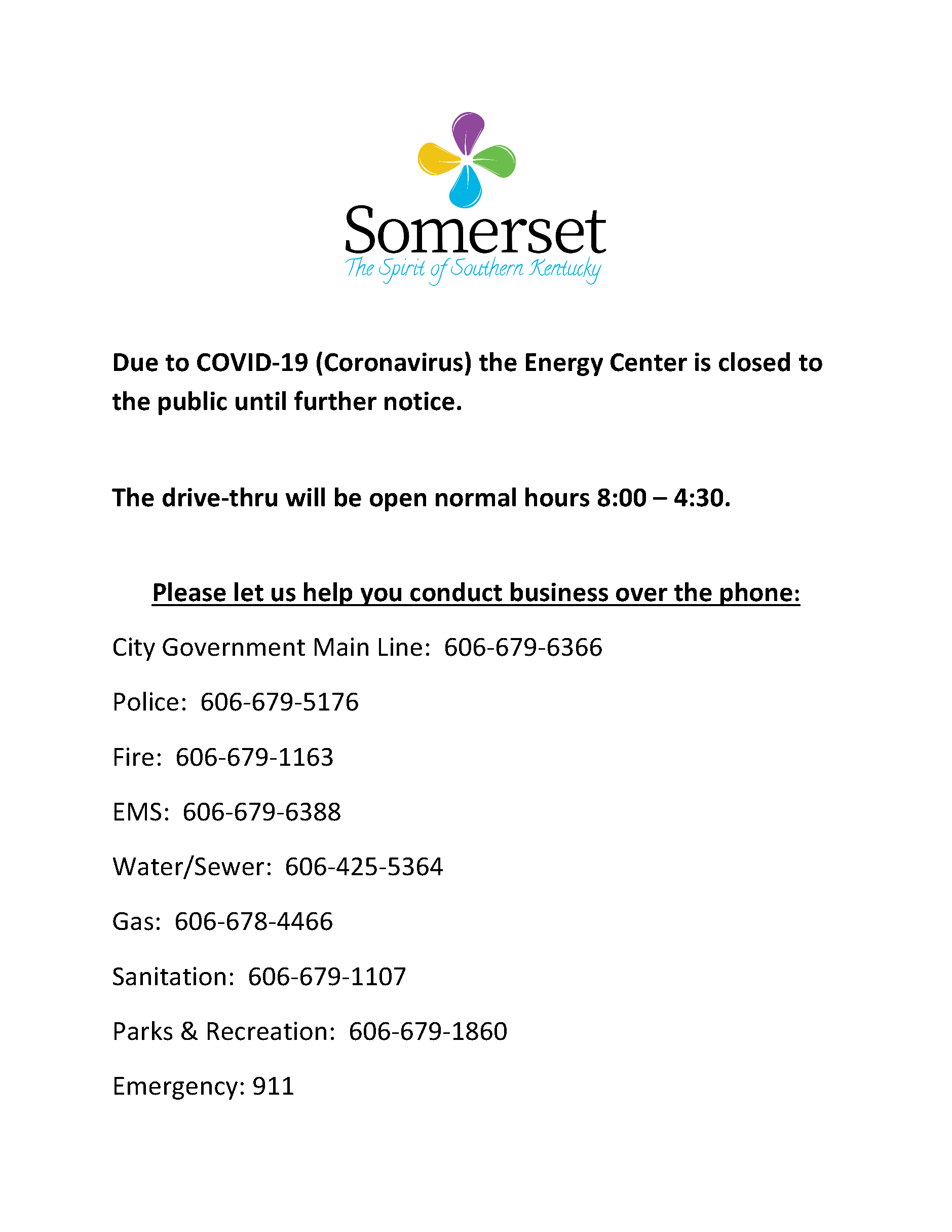The image features a vibrant drawing of a flower positioned at the top. The flower has four distinct petals arrayed in a clockwise manner starting from the top, with the petals colored in purple, green, blue, and yellow respectively. Below the flower, the word "Somerset" is prominently displayed in black, uppercase letters. Directly underneath, in elegant blue cursive font, reads the phrase "The Spirit of Southern Kentucky."

A notice follows, indicating the impact of the COVID-19 pandemic on local services:

"Due to COVID-19, the Energy Center is closed to the public until further notice. The drive-thru remains open with normal operating hours from 8:00 AM to 4:30 PM. We urge you to conduct business over the phone. 

For assistance, please contact the following numbers:

- Kentucky Government Main Line: 606-679-6366
- Police: 606-679-5176
- Fire: 606-679-1163
- EMS: 606-679-6388
- Water/Sewer: 606-425-5364
- Gas: 606-678-4466
- Sanitation: 606-679-1107
- Parks and Recreation: 606-679-1860
- Emergency: 911"

This comprehensive caption ensures clarity and provides essential contact information for various local services.